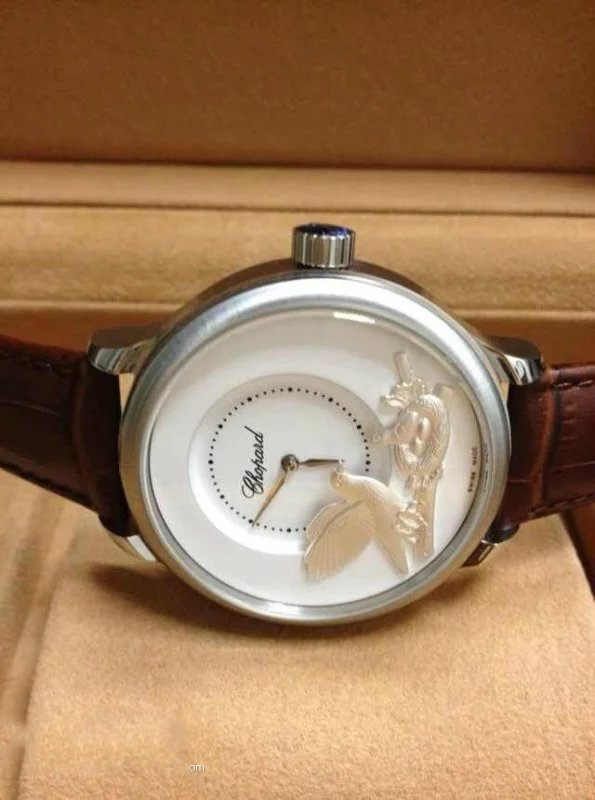The image features a watch placed against a wooden or cardboard backdrop, lending a rustic ambiance to the composition. At the center of the image, the watch stands out with its polished silver casing. On either side, there are small knobs used to adjust the hands of the watch. The watch is displayed on a leather band with a cloth underneath for support. The face of the watch is white, adorned with text and dotted markers indicating seconds and minutes. The hour and minute hands are prominent, contrasting with the minute dots. Adding a touch of elegance, the watch face features an intricate illustration of a bird perched on a tree branch.